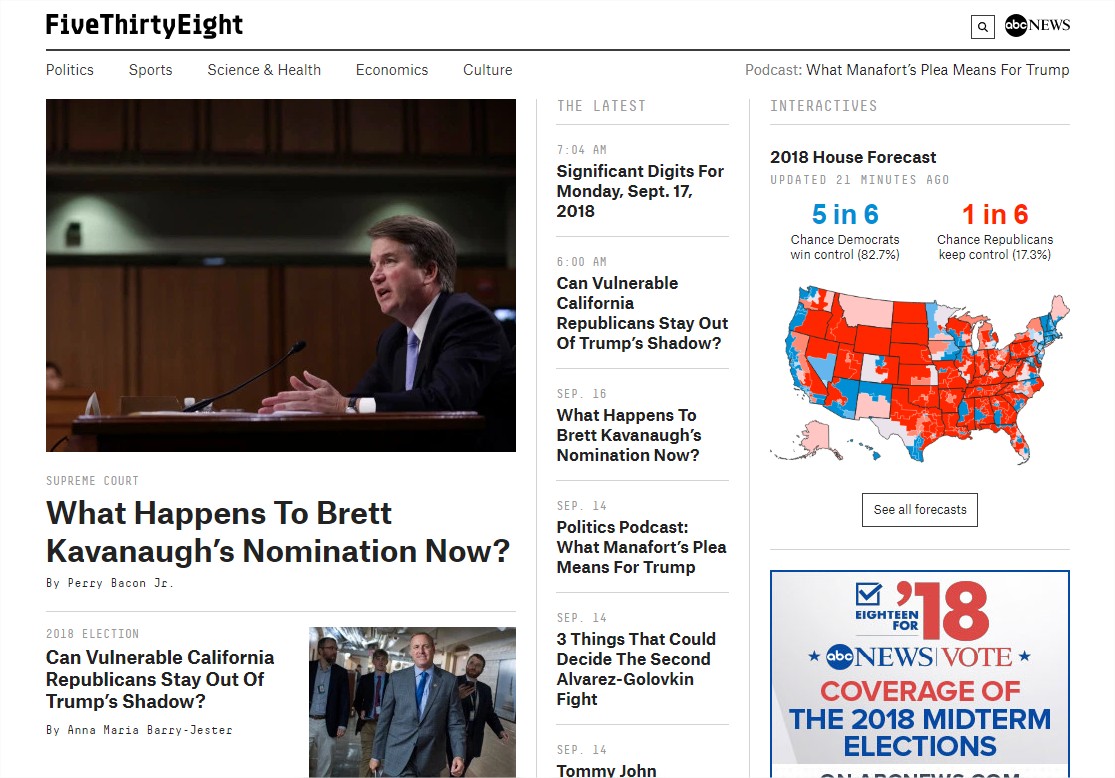Screenshot of 538 Homepage:

The webpage features a clean, white background. At the top left corner, the number "538" is prominently displayed in bold black letters. In the top right corner, there is a small square icon featuring a magnifying glass, signifying the search function. Directly next to it, the ABC News logo is visible. A slender black line separates the header from the main content.

Located directly below this black line on the left are menu categories in small black text: "Politics," "Sports," "Science and Health," "Economics," and "Culture." A large square photo occupies a central position, accompanying an article. Below the image, "Supreme Court" appears in small gray letters, followed by the bold black headline, "What Happens to Brett Kavanaugh's Nomination Now?" The article is credited to "By Terry Bacon," with the corresponding page number indicated beneath the author’s name.

Underneath this featured article, there's another story categorized under "2012 Election" in small letters. Below this, the story’s headline is displayed prominently.

In the center of the page, a vertical list titled "The Latest" begins with a date at the top and continues with a series of headlines. 

On the right side of the page, there is a vertical section labeled "Interactives," showcasing the "2018 House Forecast," which includes a map.

At the bottom right of the webpage, an advertisement promotes ABC News' coverage of the 2018 midterm elections.